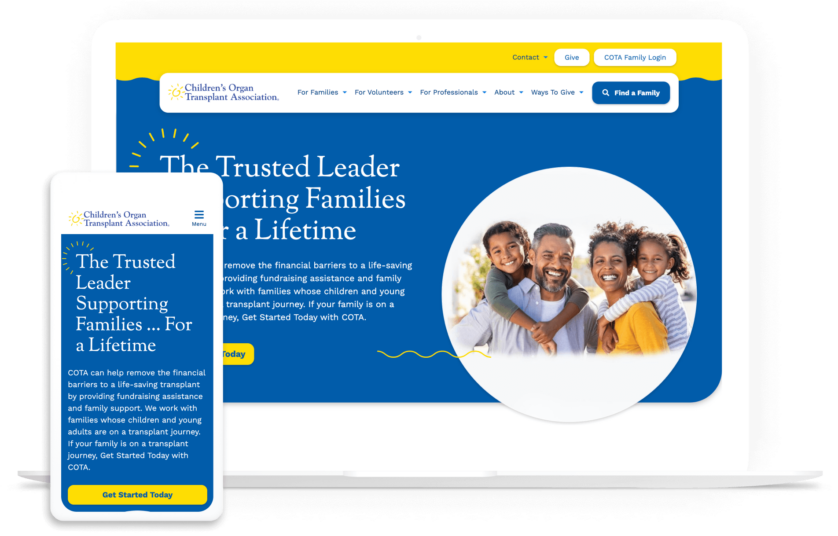The image displays a webpage from the Child Organ Transplant Association (COTA). In the top left corner, "Child Organ Transplant Association" is prominently featured in blue text, accompanied by a yellow sun icon to its left. Adjacent to this, various website categories are listed: "For Families," "For Volunteers," "For Professionals," "About," "Ways to Give," and finally, "Find a Family" highlighted in white text on a blue background in the top right corner.

Just above this section, two more options are visible: "COTA Family Login" and "Give," with a contact icon and a downward arrow to the left of "Give." Central to the webpage, the tagline "The Trusted Leader Supporting Families for a Lifetime" is displayed. 

In the bottom right, a circular image captures a family of four comprising a husband, wife, and their two children. The husband is depicted wearing a white shirt layered with a grey outer shirt, while the wife dons a yellow long-sleeved top. On the bottom left, there is an image resembling a mobile phone screen that mirrors the website, showcasing the same tagline: "The Trusted Leader Supporting Families for a Lifetime."